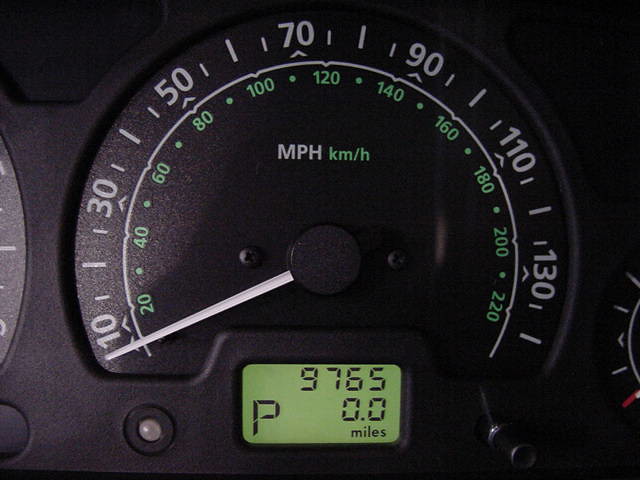The image showcases the speedometer on the dashboard of a vehicle, which features a predominantly black backdrop. The speedometer is circular with a flattened bottom, adorned along its edge with numerical markings and lines. At the center, there is a small circle with a white needle extending outwards to indicate the vehicle’s speed. Below the speedometer, a green digital screen displays the numbers "9765," followed by "0.0," and then the letter "P" for park, with "miles" situated at the far right corner. Adjacent to the screen on the left is an unlit light bulb indicator.

The primary speed indicator marks speeds of 10, 30, 50, 70, 90, 110, and 130 mph, with three smaller interval marks between each number. The middle mark of the three is notably taller. A white line encircles the bottom of the speedometer just below these numbers, and each numeric value is punctuated by a corresponding white arrow. Below this white line, the markers denote speeds of 20, 40, 60, 80, 100, 120, 140, 160, 180, 200, and 220 with a green dot between each.

The speedometer uses white letters for "MPH" (miles per hour) and green letters for "KM/H" (kilometers per hour). The numbers between 20 and 220 are in green, indicating kilometers per hour, whereas the white numbers ranging from 10 to 130 represent miles per hour.